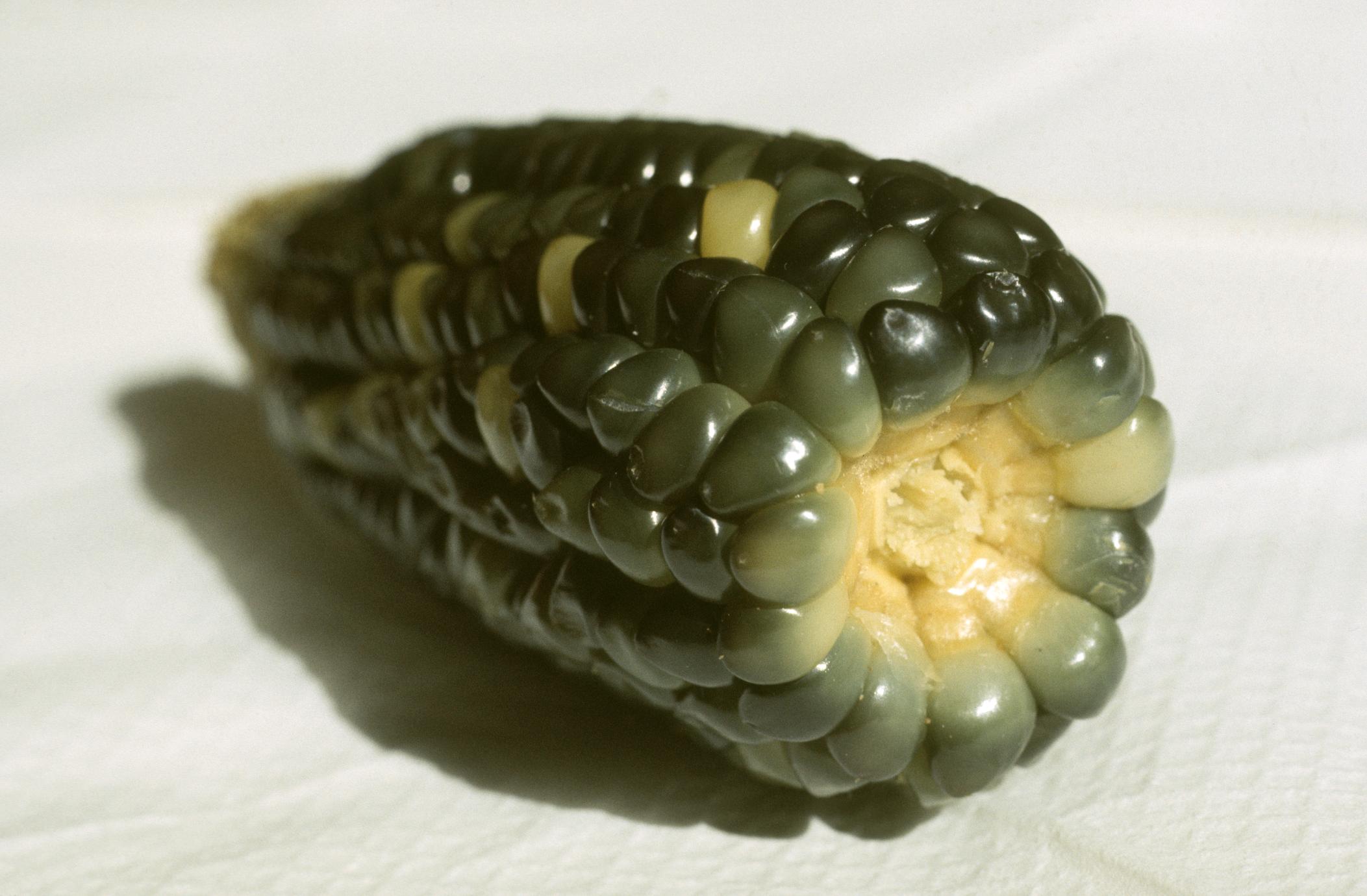This detailed photograph captures an ear of corn placed diagonally on a white cloth surface. The angle of the corn reveals both its front and side, with the base of the cob closer to the foreground and the tip in the background. The corn is unique with its dark green kernels, ranging from very dark to lighter shades, interspersed with a few rare cream-colored kernels. The core or center of the corn is cream-colored, providing a striking contrast to the green kernels. The image, taken in portrait orientation, shows the shadow of the corn falling to the left, and the background lacks any elements that would provide scale, focusing entirely on the corn itself.